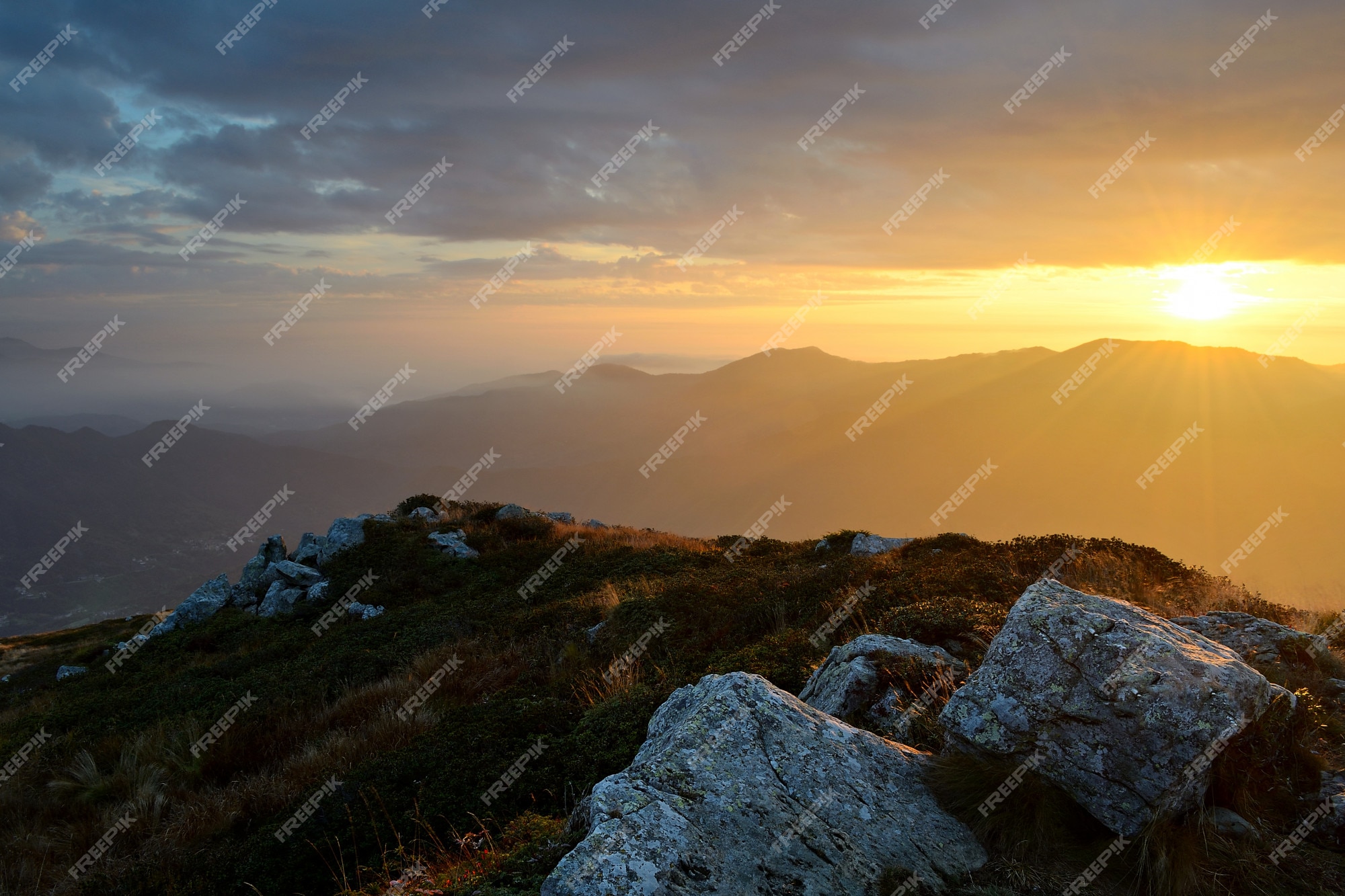This high-definition stock photograph captures a stunning mountainous landscape at sunset. The foreground, located in the bottom right corner, features prominent gray boulders surrounded by patches of green and brown grass and moss. These rocky formations extend across the lower part of the image, blending seamlessly into the rugged terrain of the mountain. As you look further into the background, a range of smoky, hazy gray mountains stretches out, adding depth to the scene. The sky above is illuminated with a beautiful mix of pink and purple hues as the sun sets, casting an amber glow over the entire landscape. Light gray, wispy clouds scatter around the sun in the upper right-hand corner, contrasting against the bright blue sky. Over the image, the watermark "Free Pik" is visible, angled at 45 degrees, appearing repeatedly in white, adding a commercial touch to this breathtaking vista.